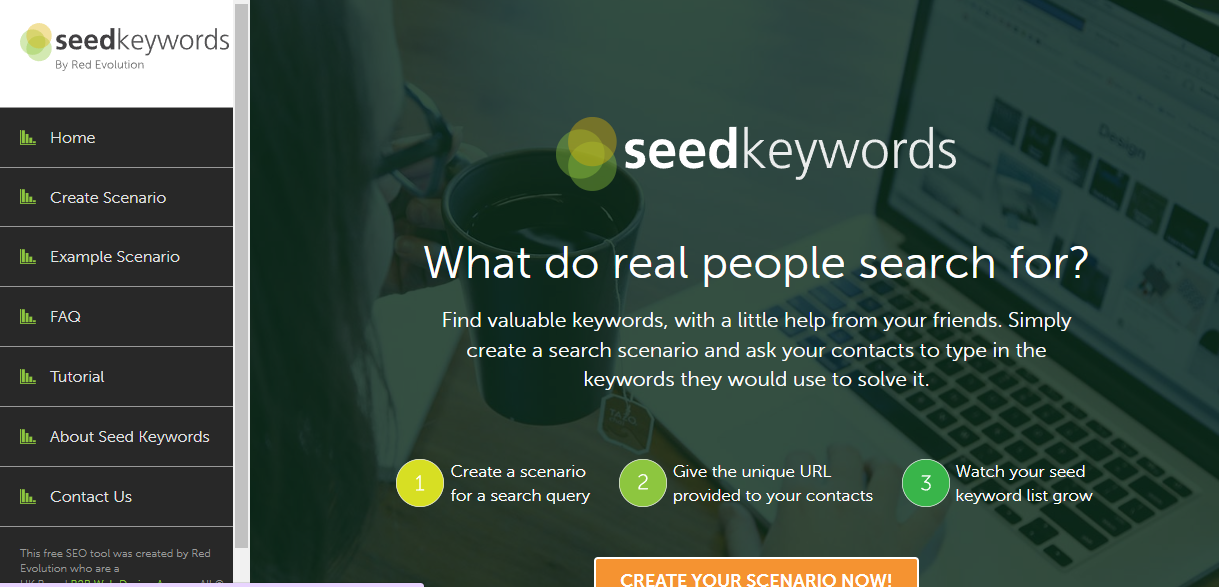**Detailed Caption:**

The web page features the "C Keywords" branding prominently across the center. The logo, marked by three interlocking circles in orange, yellow, and green, stands out, with the text "C Keywords" beside it. The “C” is highlighted in bold white, contrasting with the subtler text of “Keywords.” Beneath the logo, the slogan reads: "What do real people search for?" This tagline is followed by a concise explanation: "Find valuable keywords with a little help from your friends. Simply create a search scenario and ask your contacts to type in keywords they would use to solve it."

On the left side of the webpage, a vertical menu is present. It begins with a home button and includes sections for an "Example Scenario," a "Tutorial," and links to "C Keywords" and a "Contact Us" page.

Three steps are clearly delineated in the center of the page:
1. Create a scenario for search.
2. Share the unique URL. 
3. Watch your C Keywords list grow.

At the bottom of this instructional section, an inviting orange button features the call to action: "Create your scenario now!" The entire web page is designed to encourage users to generate real-world keyword data through collaborative search scenarios.